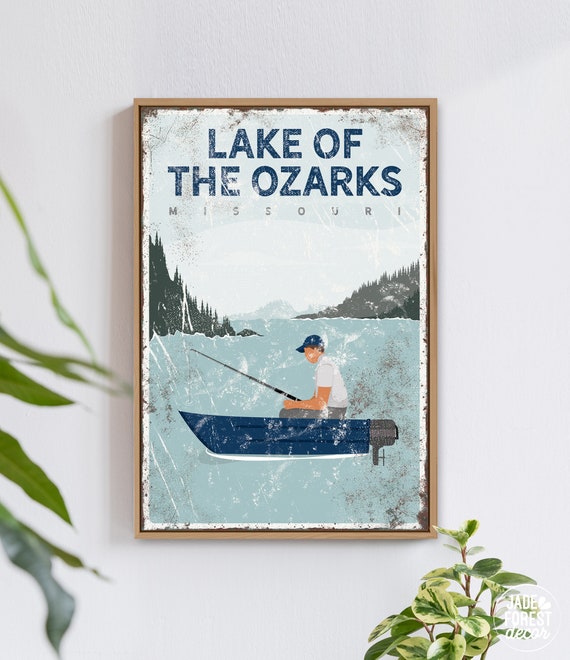The image depicts a weathered and worn painting set inside a new brown frame mounted on a white wall. The painting features text at the top that reads "Lake of the Ozarks" in bold dark blue font, with "Missouri" written in smaller print below. The scene shows a light blue lake surrounded by trees, with two mountainsides almost meeting in the center. A gentleman, wearing a white shirt, grey pants, and a blue cap, sits on a simple blue motorboat with a gray and black engine. He is holding a fishing rod. The artwork is styled simplistically, lacking intricate details or realism. Below the painting, "jade forest decor" is marked in a circle. Outside the frame, parts of plants are visible, adding a touch of greenery to the overall presentation.